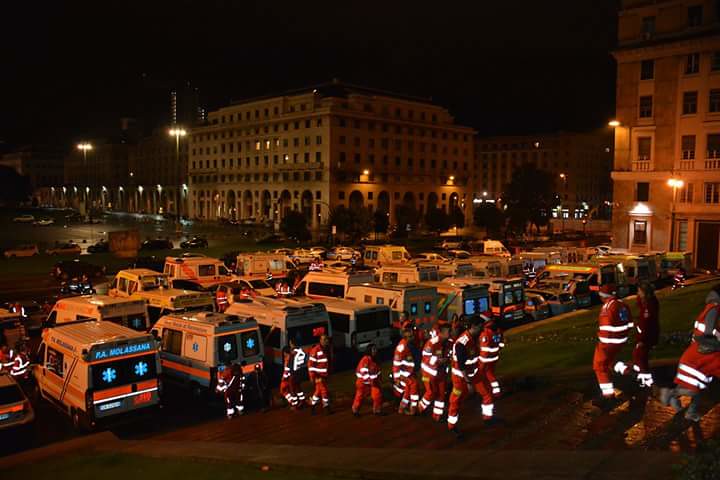In this nighttime photograph, a parking lot is densely packed with a large gathering of ambulances, both big and small, each marked with red and blue colors. A stream of emergency workers, clad in heavy orange suits with double white reflective stripes on their torsos and pant legs, is moving towards a set of stairs in the lower right-hand corner of the image. Some of these workers are seen descending from the stairs, while others are ascending, suggesting a coordinated but non-urgent activity likely reminiscent of a drill or training exercise. The backdrop features several city buildings, including a five or six-story structure, all illuminated by an array of streetlights, building-mounted lights, and tall spotlight types of lights. Additional vehicles can be observed in the distant background, further detailing this bustling city setting.